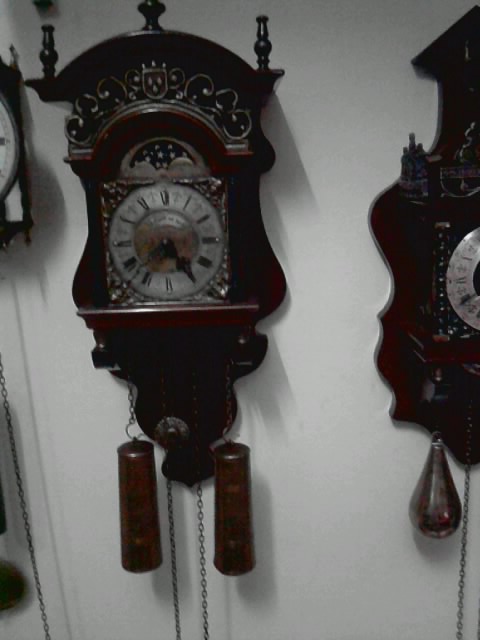The image depicts a collection of antique, old-fashioned clocks displayed on a white wall, resembling a clock store setting. At the center of the scene, an intricately carved wooden clock with a dark cherry finish stands out, showcasing a sophisticated design with Roman numerals etched onto its slightly blurred metal clock face. The time indicates approximately 5:36 or 5:37, with the hour hand on 5 and the minute hand between 7 and 8. This main clock has two wooden pendants hanging below, attached by weighted chains that dangle out of the frame.

To the right, another similar style clock is partially visible, continuing the antique theme with its own wooden carvings and dark hue, and sporting a teardrop pendant. On the left edge of the image, you can barely discern another clock, reinforcing the impression of a collection. The image has a slight motion blur, creating a sense that the photo was taken hastily, adding to the charm and authenticity of the antique setting.